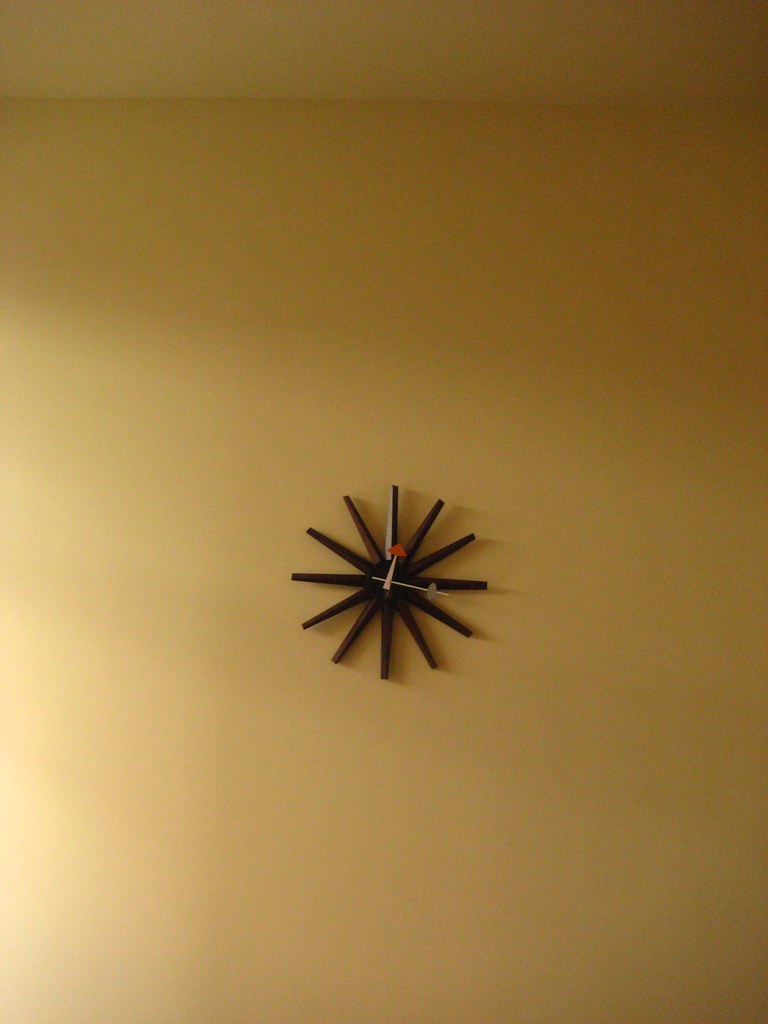In this captivating image, a highly unusual clock takes center stage against a vivid yellow wall. The clock face diverges from traditional designs, featuring a striking black starburst pattern reminiscent of an asterisk or a hand-drawn snowflake. This bold, geometric motif captures the eye, setting the clock apart from conventional timepieces.

Two distinctive hands traverse the starry expanse: the shorter hand, adorned with a small red triangle at the tip of a tan shaft, and the longer, more slender hand, marked by a green oval. These vibrant accents provide a playful contrast to the monochromatic backdrop of the clock face.

The juxtaposition of the clock's intricate design against the solid yellow background creates a visually compelling centerpiece, emphasizing the uniqueness of this time-telling work of art.